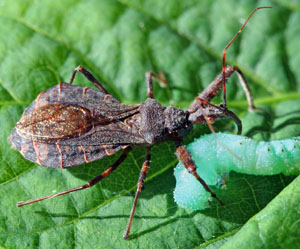The photograph features a close-up, zoomed-in image of a dark brown shield bug or stink bug, which is holding onto a small, light green caterpillar, most likely its prey. The bug is distinctly marked with yellow-orange stripes across its back and has black and orange legs, alongside prominent antennae and a visible proboscis extending from its mouth. The caterpillar is light green with noticeable body sections and tiny dots along its wrinkled skin. Both insects are positioned on a green leaf, which serves as the background, displaying its texture and veins in a different shade of green than the caterpillar. The imagery captures the moment right before the bug consumes its catch, emphasizing the intricate details and colors of the insects and their natural habitat.